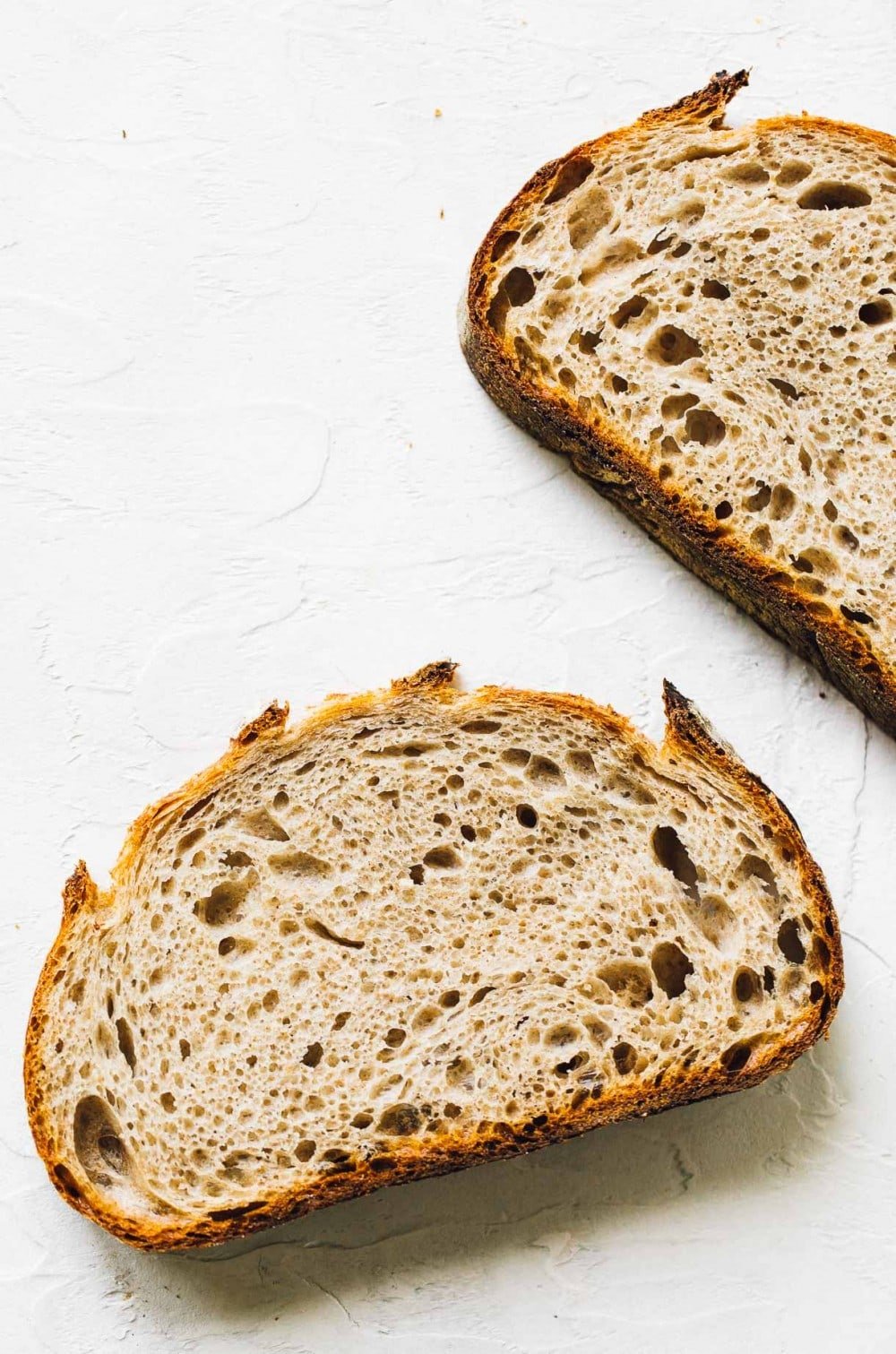The image depicts two pieces of crusty, roughly cut bread on a white table, highlighting its uneven surface. The bread has a bright brown, chewy crust, indicating it was likely recently baked. The inside contains numerous small nooks and crannies, reminiscent of an English muffin, suggesting the presence of oxygen bubbles. The first piece of bread sits at the bottom of the frame, tilted slightly upward, while the second piece is positioned at the middle top, also tilted upward. The overall color palette includes beige and brown tones, reflecting the toasted appearance of the crust and the natural color of the bread's interior. This bread appears to be from a small, rounded loaf, and not intended for typical sandwich use, as it is thickly cut and hearty in texture.